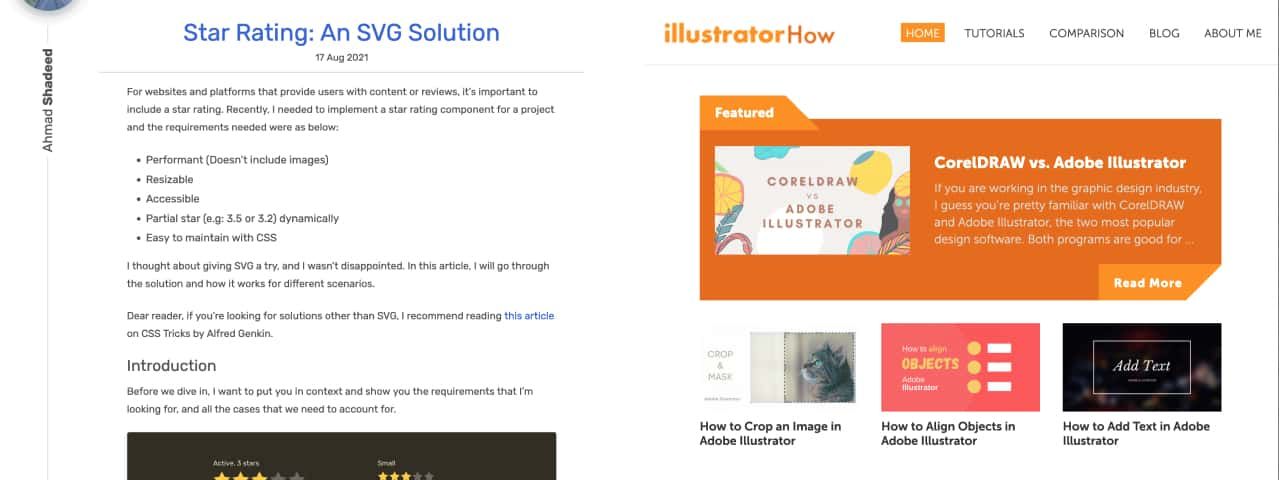The image is a screenshot of a website featuring varied content related to graphic design and star rating implementation. The background of the page is predominantly white, accentuated with text in shades of black, orange, and blue.

On the left side of the image, the blue heading reads "Star Rating and SVG Solution," followed by a subheading in black that states "17th of 2021." It explains the importance of incorporating a star rating system for websites and platforms that provide user content and reviews. The author shares that they needed to create a star rating component for a project, outlining the requirements: usefulness without images, resizable for different contexts, accessibility compliant, partial star capability, dynamic functionality, and ease of maintenance with CSS. The author opted to explore an SVG-based approach and found it satisfactory. The article details this solution, its applicability in various scenarios, and suggests an alternative reading on CSS tricks by Alfred Gecken for those interested in non-SVG solutions.

Below this section, there is a prominent, neatly bordered brown box displaying several star icons.

On the right side of the image, in bold orange text, it reads "Illustrator How," accompanied by a navigation bar with options: "Home" in orange and white, followed by "Tutorials," "Comparison," "Blog," and "About Me" in black. 

Further down is a large orange box with a white text banner and an image titled "Coral Draw vs. Adobe Illustrator" in a salmon color. The image contains visuals of oranges and a feather, alongside a cartoon depiction of a dark-skinned woman. Below the title, it elaborates briefly on the familiarity and popularity of these design software applications within the graphic design community. The text trail off with an invitation to "Read More."

Additionally, the page has a section featuring three smaller images at the bottom, each with accompanying black text: 
1. A brown cat with the caption "How to Crop an Image in Adobe Illustrator."
2. A salmon, gold, and white graphic, titled "How to Align Objects in Adobe Illustrator."
3. A black and white box labeled "Add Test," with a description reading "How to Add Text in Adobe Illustrator."

This screenshot effectively encapsulates various aspects of the website, targeting both star rating implementation and graphic design software comparisons and tutorials.